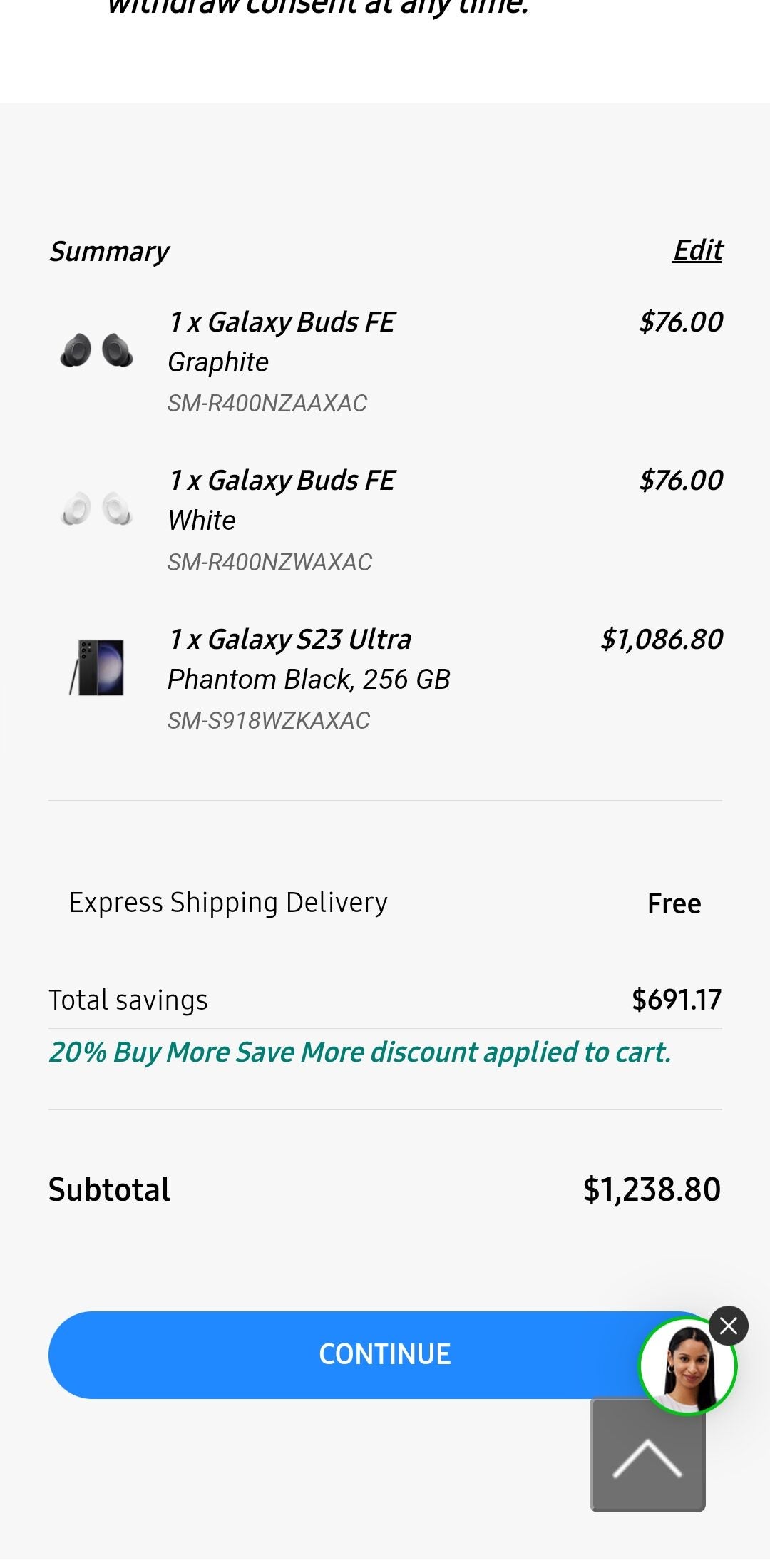Here is a refined and detailed caption:

---
The image displays a detailed sales receipt summary. The first row showcases an image of each purchased product, followed by their respective names in the second row. The third row lists the prices. Specifically, the receipt indicates the purchase of three items: one pair of Galaxy Buds FE in graphite color, another pair in white, and a Galaxy S23 Ultra in Phantom Black with 256GB storage. The listed prices are $76 each for the Galaxy Buds and $1,086.80 for the Galaxy S23 Ultra. An express shipping option is noted as free. Additionally, the buyer has saved $691.17, with a special "20% Buy More, Save More" discount applied to the cart, resulting in a subtotal of $1,238.80. At the bottom of the receipt, there is a blue 'Continue' button, and on the right side of the image, a profile picture of a woman with long black hair is shown.